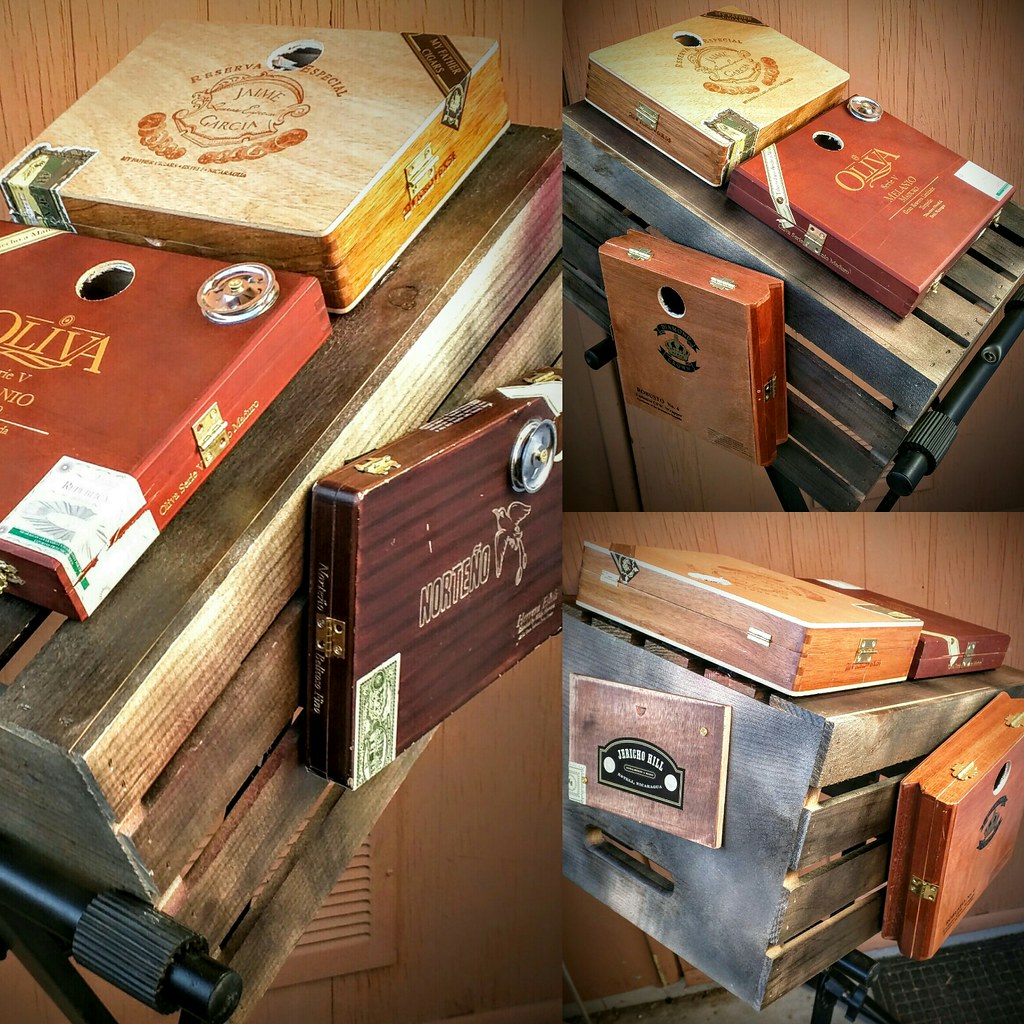An image collage depicts a wooden crate from multiple angles. The left side features a single image showing a wooden crate with two old books atop—one with a red cover and another with a white cover. Adjacent to the crate is a small box. A black stand supports the crate, and the background consists of wooden planks.

The right side of the collage comprises two smaller images stacked vertically. The upper image presents a frontal view of the same crate, which now shows a blue-tinted front edge. The books atop the crate are identical but slightly different in color due to the angle. The lower right image offers a side view of the crate, revealing additional details of the books and another wooden case beside the crate.

Each box attached to the crate is about the size of a briefcase, equipped with metal hinges and small holes. The boxes bear inscriptions like "Oliva" (often obscured) on the red one with gold writing, "Jaime Garcia Reserva Especial" on the beige one with reddish-brown writing, and "Norteno" on the brown one with yellowish-white writing. The various angles capture different perspectives of the same setup, emphasizing the nuanced details and inscriptions on the crates and books.